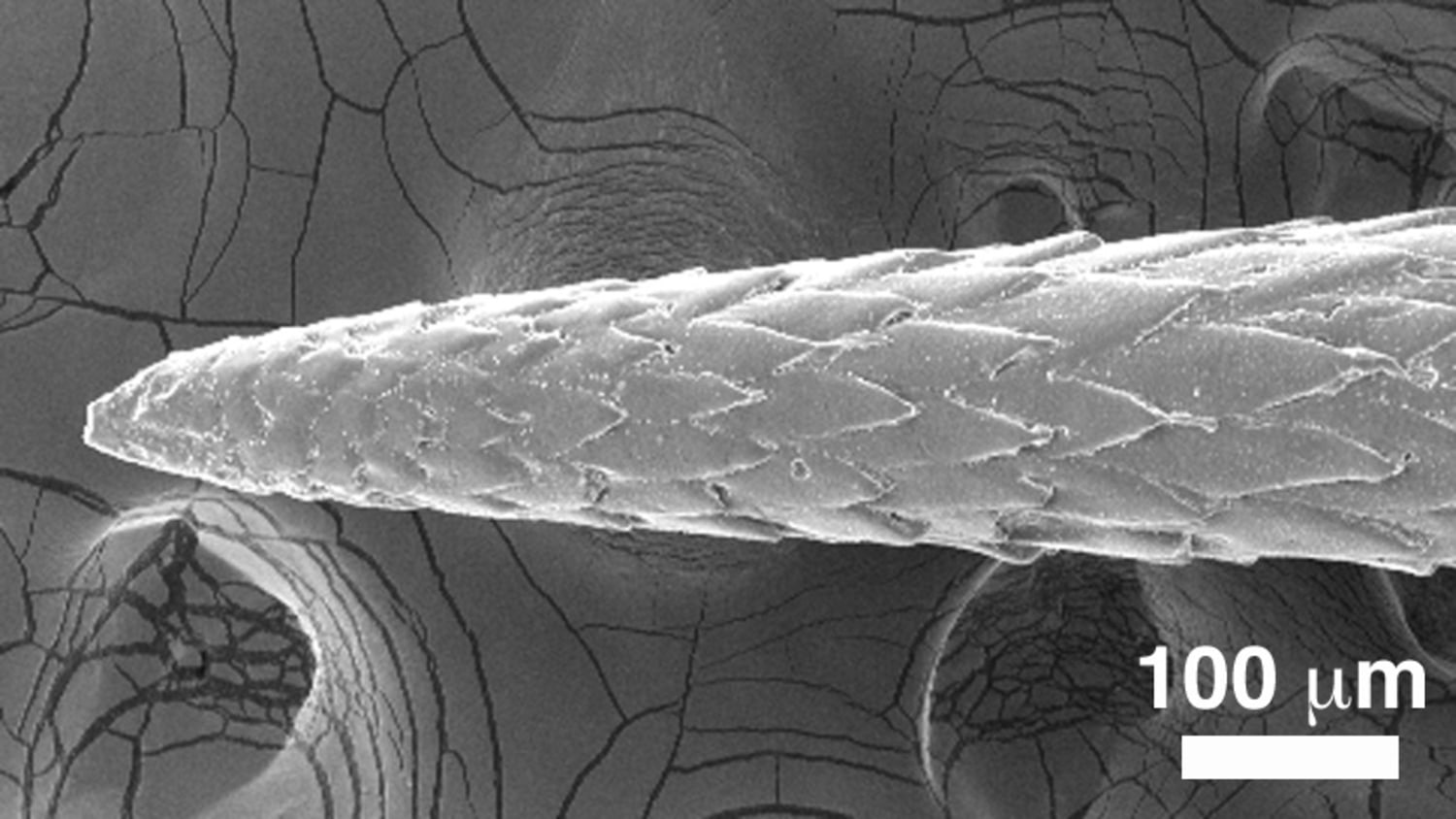The black and white photo appears to be an extreme close-up, likely taken with an electron microscope. The background is a dark gray, adorned with black lines crisscrossing it, resembling cracks or perhaps fissures. In the center of the image, a large white oval shape dominates, featuring etched zigzag patterns that give it an intricate texture. Extending from the right side of the frame, the main subject of the photo is a cone-shaped object that tapers to a point toward the left, and it is characterized by pronounced ridges along its surface. The object and the central oval are rendered in varying shades of light gray. Intriguingly, in the bottom right corner, there is a label in white text that reads "100 UM," accompanied by a horizontal white bar that extends from the first '0' in '100' to the middle of the 'M' in 'UM,' serving as a scale indicator. The presence of this 100 micrometer marker suggests that the image captures an incredibly small entity, far beyond the resolution of the naked eye.